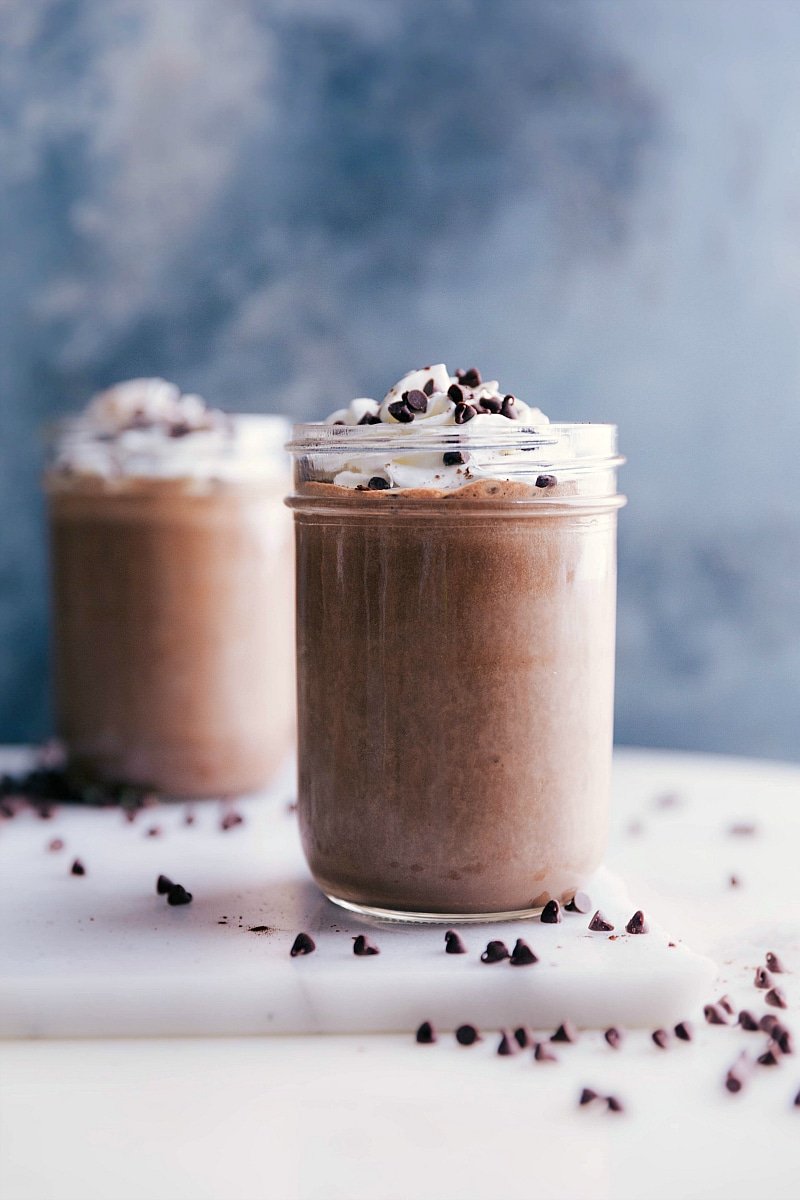This color photograph, oriented in portrait, showcases a clear glass cup filled with a rich, creamy chocolate drink positioned centrally in the frame. The glass features a screw-on lid and contains a brownish, frothy beverage topped with a generous dollop of whipped cream. Dark chocolate chips are scattered over the whipped cream and also around the cup on the white marble rectangle surface it sits on. Behind this focal drink, slightly out of focus, is another identical chocolate drink placed to the left. The backdrop is an abstract blue and white pattern resembling a sky with clouds, enhancing the visual appeal of the scene. The image, characterized by photographic representationalism and realism, exemplifies meticulous food photography.